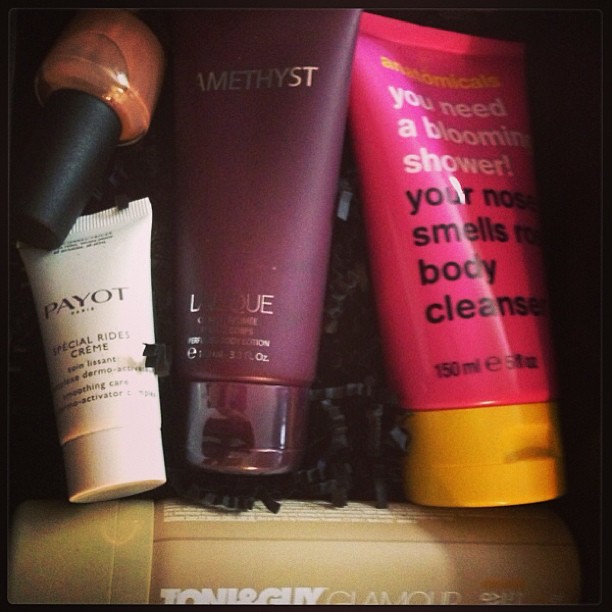In a dimly lit setting, possibly inside an open drawer or on a shelf, four inverted beauty products are prominently displayed, illuminated by a focused light source. Starting from the right, there is a large pink tube with a yellow cap. It reads "You Need a Blooming Shower," followed by "Your Nose Smells" and "Body Cleanser," alongside "150 mg" in white lettering. Next to it is a dark purple tube with a reflective cap, marked "Amethyst" in silver lettering. While the manufacturer is partly obscured, it appears to say "Lalique." To its left is a smaller white tube labeled "PAYOT" with additional text identifying it as "Special Ridge Cream." Completing the lineup, at the top left, is a bottle with a cylindrical black cap, filled with a rust-colored liquid, possibly nail polish or makeup. All products are neatly arranged, providing an organized yet intimate glimpse into a collection of personal care items.